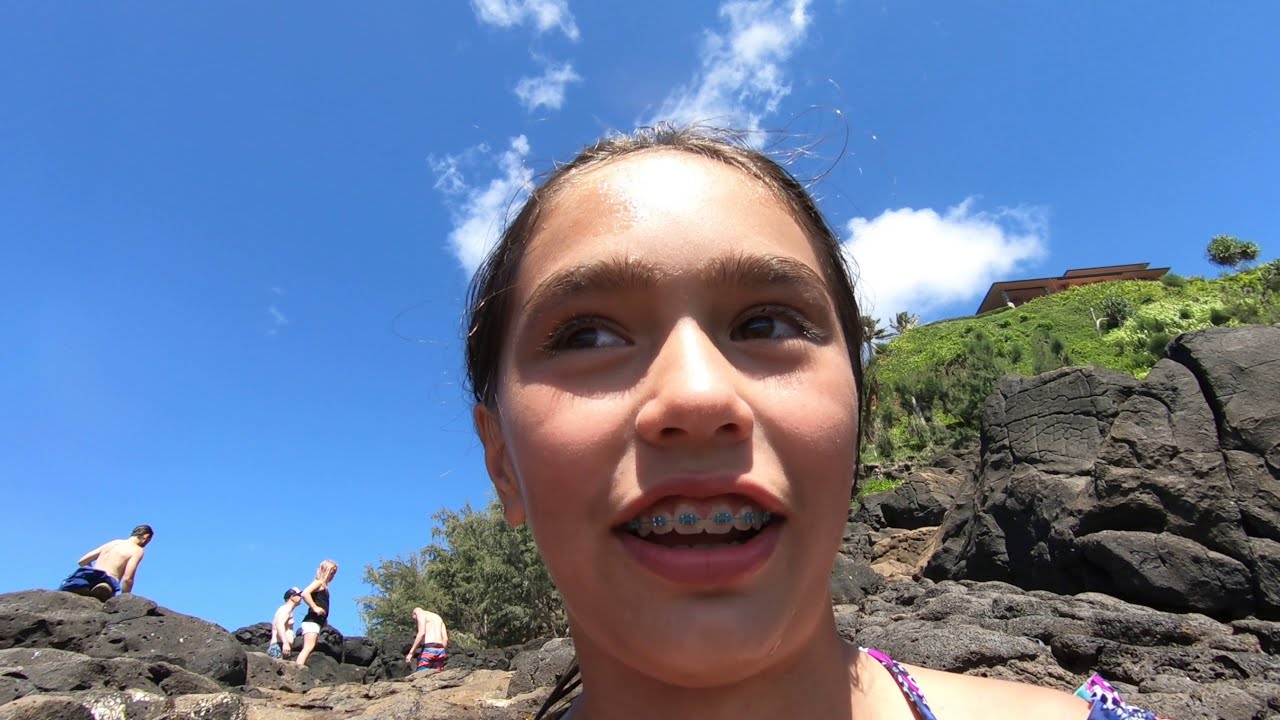This vibrant photograph captures a young girl, estimated to be around 13 or 14 years old, smiling and looking off to the left. The girl, who is wearing braces and has her hair pulled back, is positioned directly in the center of the image, drawing immediate attention to her joyful expression. She appears to be wearing a top that ties at the back, possibly indicating she is dressed for swimming.

In the background, standing on the rocky cliffs, are several people, including a girl of similar age wearing a black tank top and white shorts, and three shirtless men in swim trunks, indicating a casual, beach-like setting. The men are variously dressed in pink and blue swim trunks, blue swim trunks, and one even has a white and blue baseball hat on.

The rocky cliffs surrounding them are distinctive, with steep, lava rock formations and sparse vegetation, including patches of green grass and some bushes and small trees higher up. To the top right of the image, a house is nestled among palm trees, suggesting a tropical island location. Above this scene, the sky is visible, dotted with some clouds, emphasizing the outdoor, midday setting of this photograph. This vivid snapshot captures a moment of leisure and natural beauty, devoid of any text, allowing the scene to speak for itself with its colorful palette of blue, white, gray, tan, black, and purple hues.